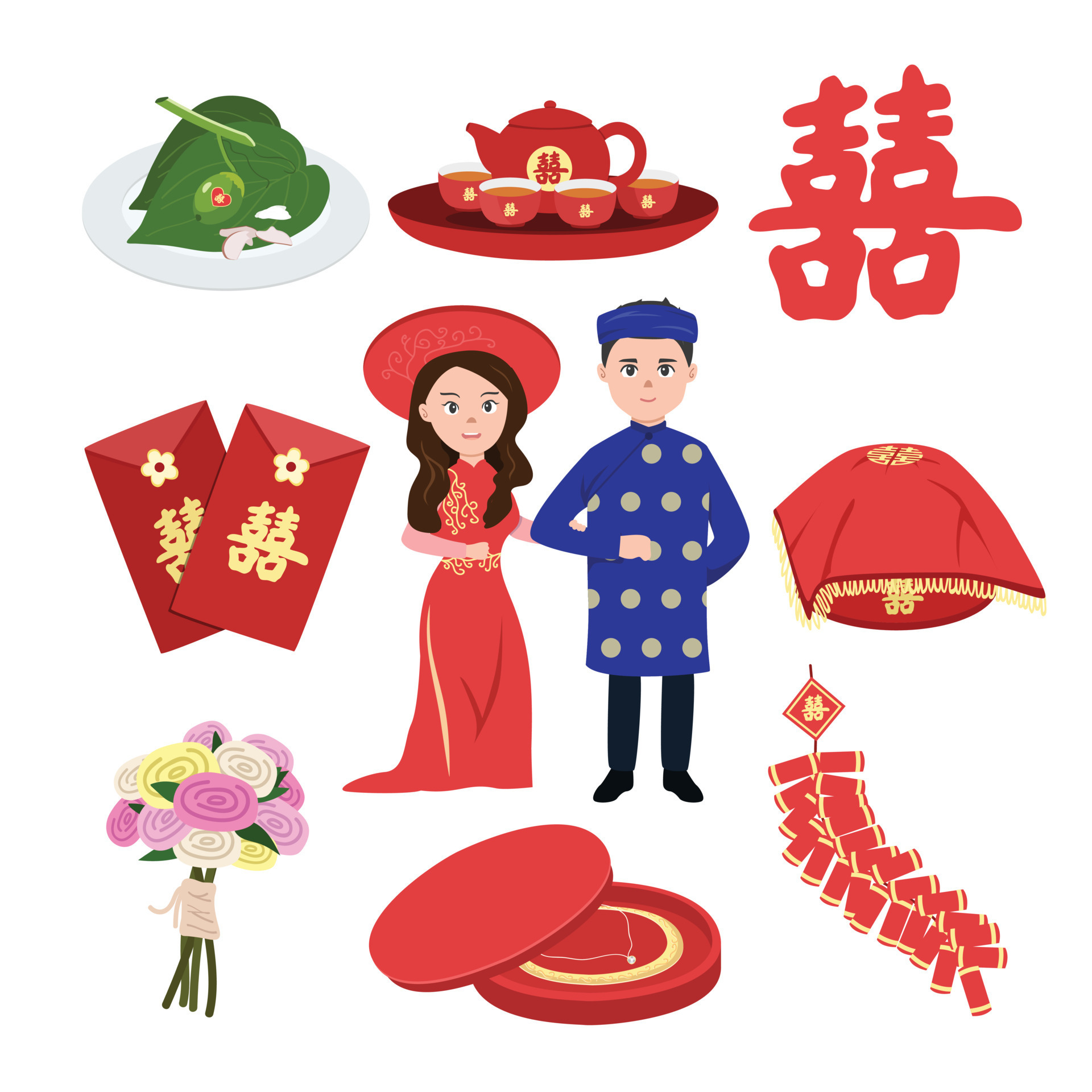The image is an intricate drawing featuring a collection of Asian-inspired graphics that collectively suggest a Chinese celebration, possibly a wedding or tea ceremony. Central to the composition is a couple in their 20s; the woman, with long dark hair and brown eyes, wears a vibrant red, short-sleeved cultural outfit adorned with gold details and a matching large red hat. She stands arm in arm with a man dressed in a long blue garment with greenish dots, a matching blue hat, black pants, and black shoes.

Surrounding the couple are multiple festive elements: 

- **Top Left**: A red plate displaying green leaves and white items resembling spices. 
- **Top Center**: A traditional red tea set comprising a red and gold teapot with Chinese symbols, accompanied by four red cups also bearing Chinese symbols.
- **Top Right**: A prominent red Chinese symbol.
- **Middle Left**: Two red envelopes with gold Chinese symbols and floral seals.
- **Middle Right**: A decorative red pillow with gold embellishments and Chinese writing, with gold loops around its rim.
- **Bottom Left**: A colorful bouquet featuring pink, yellow, purple, and white flowers wrapped in a cream-colored ribbon.
- **Bottom Center**: A red box containing a delicate necklace with a thin chain and a central stone, possibly a diamond.
- **Bottom Right**: A series of red and gold firecrackers.

The entire collage, set against a white background, is a harmonious blend of traditional Chinese motifs rendered in vibrant red and gold hues, emphasizing the celebratory and auspicious themes associated with Chinese culture.